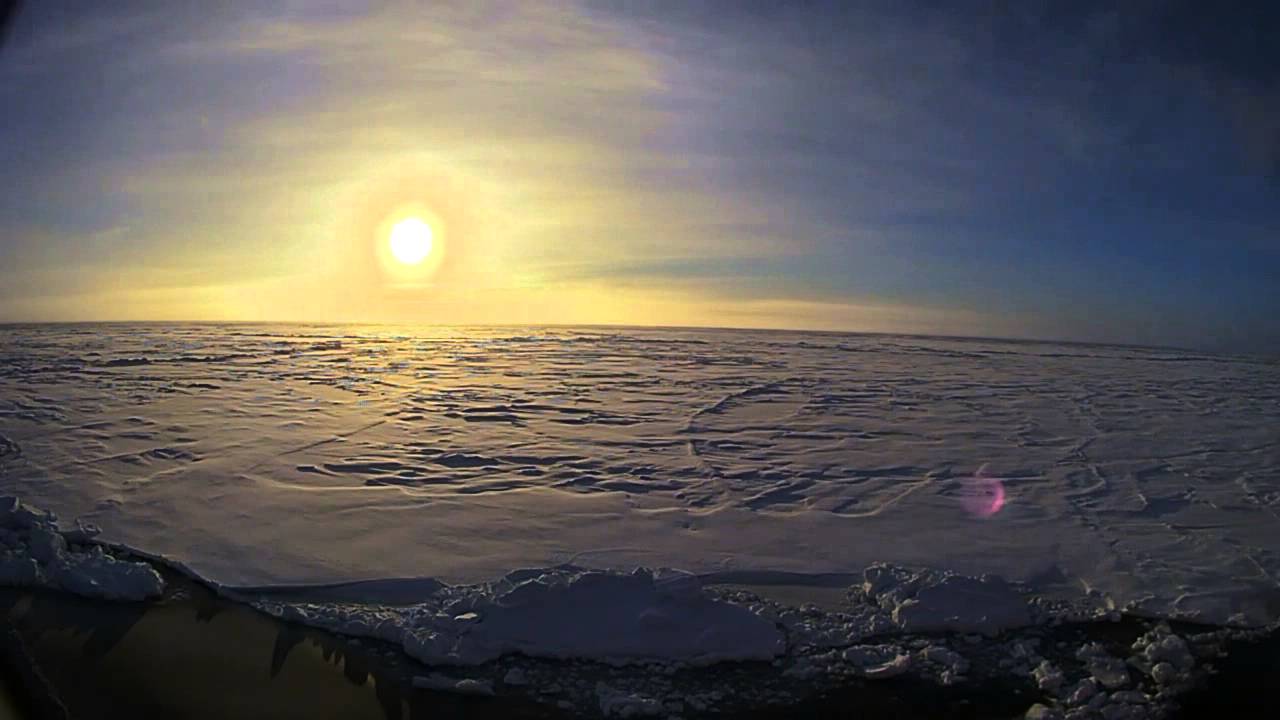This image captures a captivating sunset over a frozen sea, where the sun is just a little above the horizon. The golden yellow light from the setting sun radiates outward, transitioning the sky from light blue near the horizon to darker shades of blue towards the edges. The ground, which appears to be a mix of wet sand, smooth rocks, and ice, forms a horizontal band across the middle of the frame. This frozen expanse is sometimes smooth, sometimes ruffled, possibly due to wind. Reflections on the ice create intriguing visual elements, including a round, purple transparent circle and what seems to be a rectangle resembling a cherry. The frozen sea is intermittently covered with snow and ice fragments, adding texture to the otherwise serene and chilling landscape.